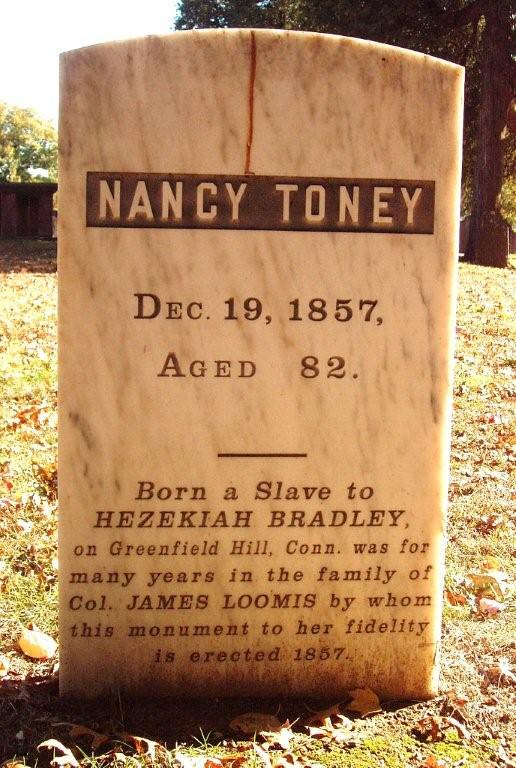This image depicts a memorial tombstone, rectangular with a curved top, situated outdoors in a graveyard. The tombstone is crafted from marble and is engraved with block letters that read "Nancy Toney." Below her name, it states "December 19, 1857, aged 82." There is a horizontal line separating this text from the subsequent inscription: "Born a slave to Ezekiel Bradley on Greenfield Hill, Connecticut, was for many years in the family of Colonel James Loomis, by whom this monument to her fidelity is erected, 1857." The tombstone, brown in hue, is surrounded by green grass scattered with a variety of leaves. In the backdrop, there is a tree and several other monuments visible in the distance, contrasting with the lush grassy expanse.